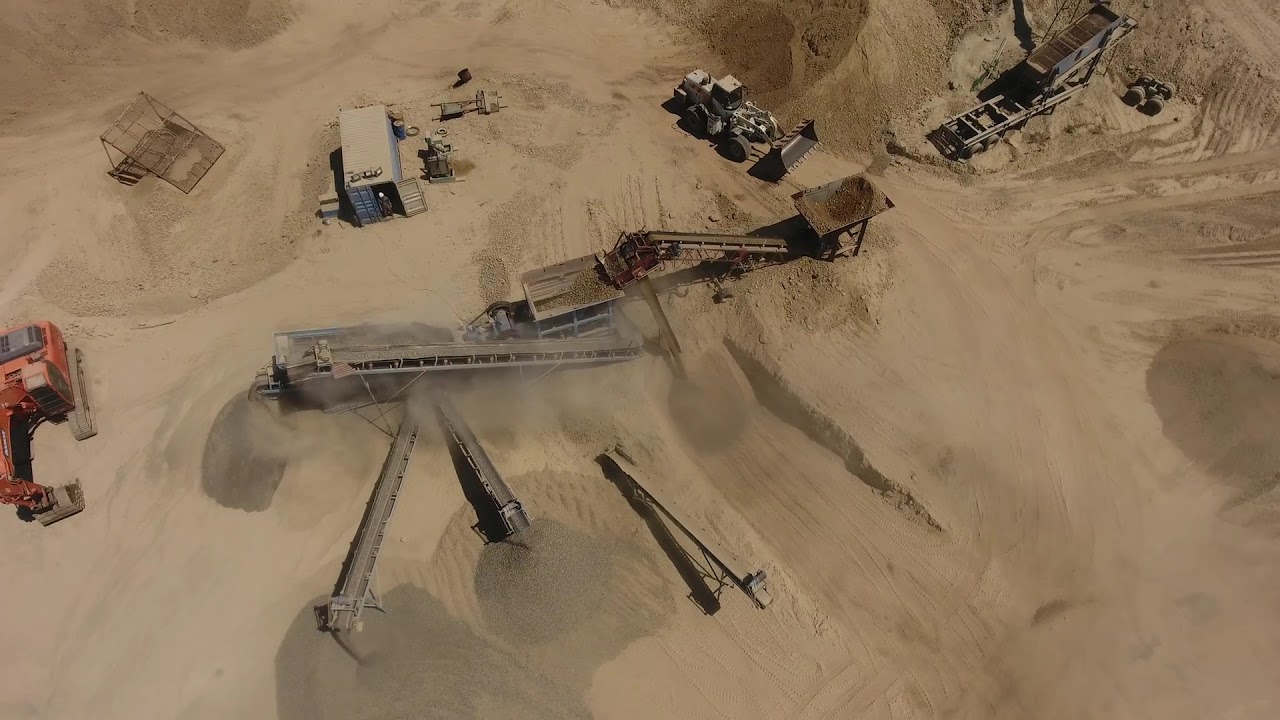This aerial photograph captures a sprawling construction or mining site, predominantly composed of light brown sand. The scene is dotted with various large pieces of mobile equipment, notably bulldozers and vehicles on caterpillar treads. Dominating the left side of the image is a red bulldozer next to a blue cargo container, from which a man in dark clothing and a white hard hat stands in the doorway, surrounded by miscellaneous items. Adjacent to the container is a gray bulldozer with its scoop lowered, working alongside a conveyor belt, part of a network of belts scattered throughout the site. These conveyor belts are actively transporting and piling sand. The bright daylight illuminates the entire sandy expanse, where machinery and ramps are seen working randomly to process ore or other construction materials, contributing to a bustling industrial environment.